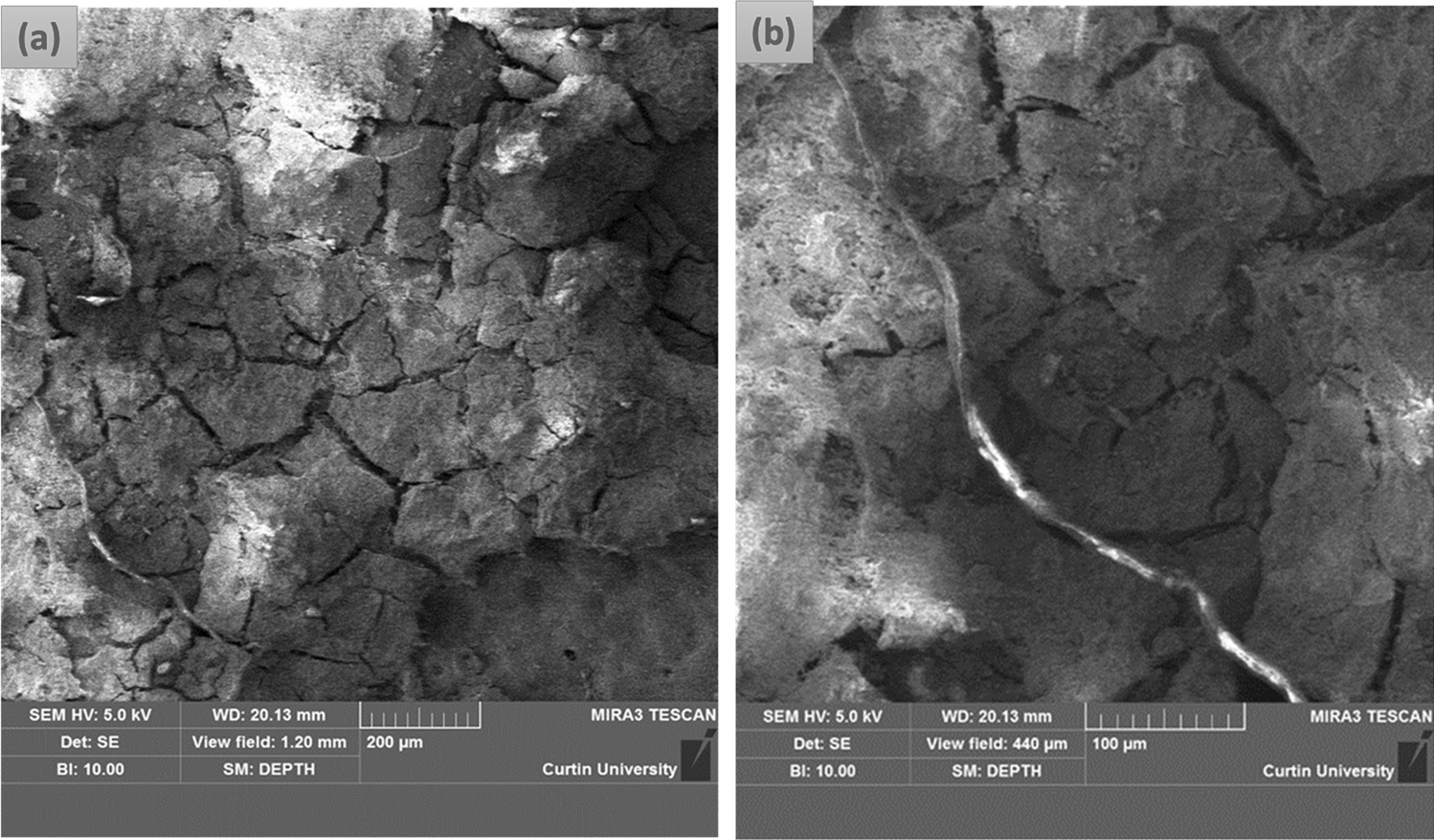This black-and-white photograph, possibly taken from a satellite or a high-resolution camera, displays two side-by-side images labeled A and B. Each image reveals cracked, gray rock, with the right image (B) distinctly showcasing a prominent fissure. Detailed technical annotations are inscribed below both images. For image A, the text reads "SEMHV 5.0 KV DET SE BL 10.00 WD 20.13 mm view field 1.20 mm SM depth MIR A3 TESCAN CURTIN CURTIN University," while for image B, the view field measurement is "440." Both annotations feature "MIR A3 TESCAN CURTIN University," suggesting an affiliation with Curtin University. The entire setup, with its fine details and high level of precision, seems to originate from a university-related probe or imaging device capturing the rugged terrain for scientific analysis.